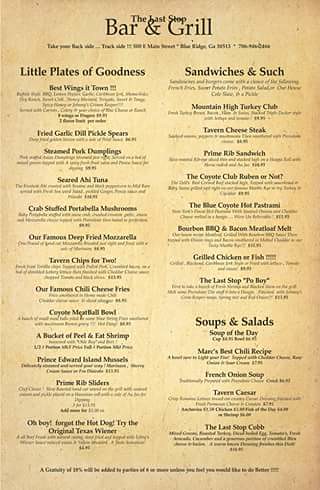Indoor color close-up photograph of a visually appealing menu page from a restaurant. The top of the menu features the phrase "The Last Stop" in small print, followed by the establishment's name, "Barn Grill," in prominent green lettering. The menu is organized into two distinct columns, each with various categorized sections.

On the left column, the heading "Little Plates of Goodness" stands out, listing approximately 20 delectable dishes. A few notable items under this section include “Buffalo Wing It Town,” “Fried Grilled Dill Pickle Spears,” an indecipherable entry, and “Tavern Chips for Two.”

The right column similarly features categorized subsections. The first heading reads “Sandwiches and Such,” under which around seven to eight sandwich options are listed. Following this, the section “Soups and Salads” appears in the lower right corner, offering about four selections.

The menu is designed to look vintage, with a deliberately aged paper appearance, adding to its charm, though it remains in pristine condition with no visible tears or rips.